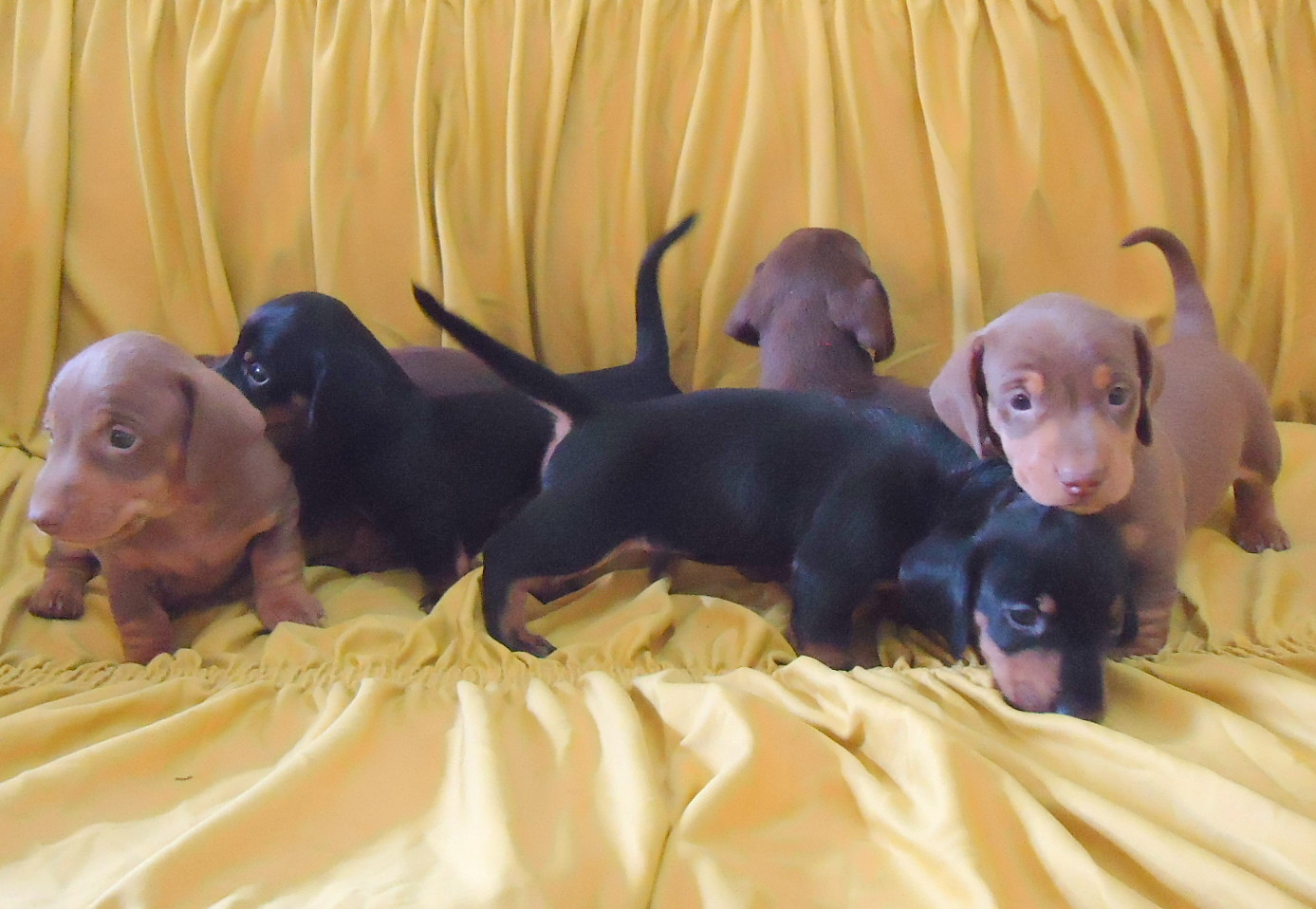This photograph showcases a group of five adorable puppies, possibly Dachshunds or a mix of similar breeds, gathered on a ruched lemon-yellow fabric background. The scene suggests an energetic and slightly restless group, as indicated by their varied poses and animated tails. Three of the puppies are light brown with tan markings on their chest, muzzle, and paws, giving them a distinct appearance. The other two resemble Rottweilers or German Shepherds, displaying black coats with tan accents around their chins, undersides, and paws. 

Among the group, one black and tan puppy is positioned at the front, facing towards the right, while another of the same color looks to the left. The three light brown puppies are dispersed around them, with one on the far right gazing directly at the camera, exuding a curious demeanor. Another, situated in the background, has its head turned away, seemingly uninterested in the photo session. The third light brown puppy is on the far left, looking off to the left with inquisitive eyes. Overall, these playful pups, surrounded by the vibrant yellow backdrop, create a lively and heartwarming snapshot.